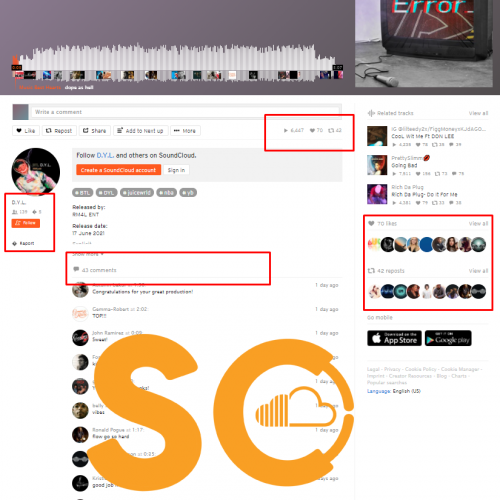This image is a screenshot of a web page interface. At the top, there is a lengthy gray rectangular bar, resembling the header section. Embedded within this header is a gray and white striped bar graph-like feature, which appears to function as a timeline, showcasing various thumbnails at its base.

Below this header, a microphone is seen lying on a gray floor, suggesting an audio-related context. Further down the page, there is an interactive section for user engagement, featuring options to write a comment, like, repost, share, and a button to "Add to Meetup." A "More" option accompanied by three dots is also present.

A user profile picture, contained within a circular frame, is visible on the left. Several red rectangular boxes highlight key areas of interest on the page, likely for emphasis in a presentation. One red rectangle is located towards the top, another just beneath the profile picture, and a longer, thinner rectangle highlights an area labeled "43 comments."

Additionally, the page includes prominent letters "S" and "O" in purple, with the "O" containing a cloud graphic, indicating some element of branding or thematic design.